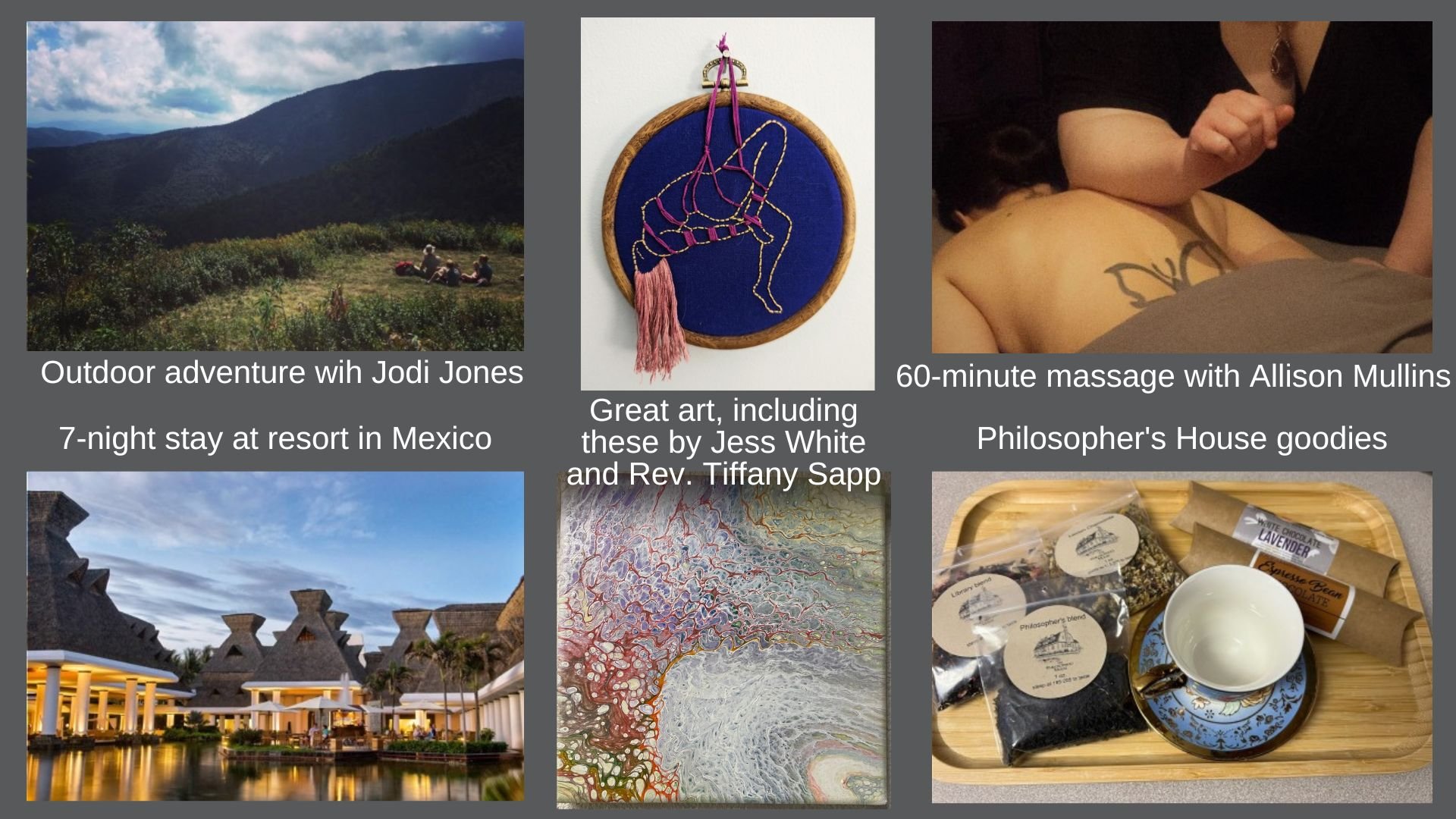This image is a promotional collage with six distinct pictures, all detailing various activities and offerings for a retreat. 

In the upper left-hand corner, there is an advertisement overlaying a scenic landscape featuring three people picnicking in a grassy field, gazing at a majestic mountain range shrouded in clouds. The caption here reads, "Outdoor Adventure with Jody Jones."

To the right of this, there's an ornate piece of embroidery art, featuring intricate gold and red patterns, attributed to "Great Art including these by Jess White and Reverend Tiffany Sapp."

Further to the right, a soothing scene depicts a person receiving a massage, captioned as "60-minute massage with Allison Mullins."

In the bottom left, an enticing offer reads "Seven-night stay at a resort in Mexico," accompanied by an image of serene cottages by the water, exuding tranquility.

Adjacent to this, an abstract painting with wavy patterns in purple and red catches the eye. 

Finally, on the far right, a quaint display named "Philosopher House Goodies" showcases a teacup and three clear bags of tea, elegantly arranged on a wooden tray.